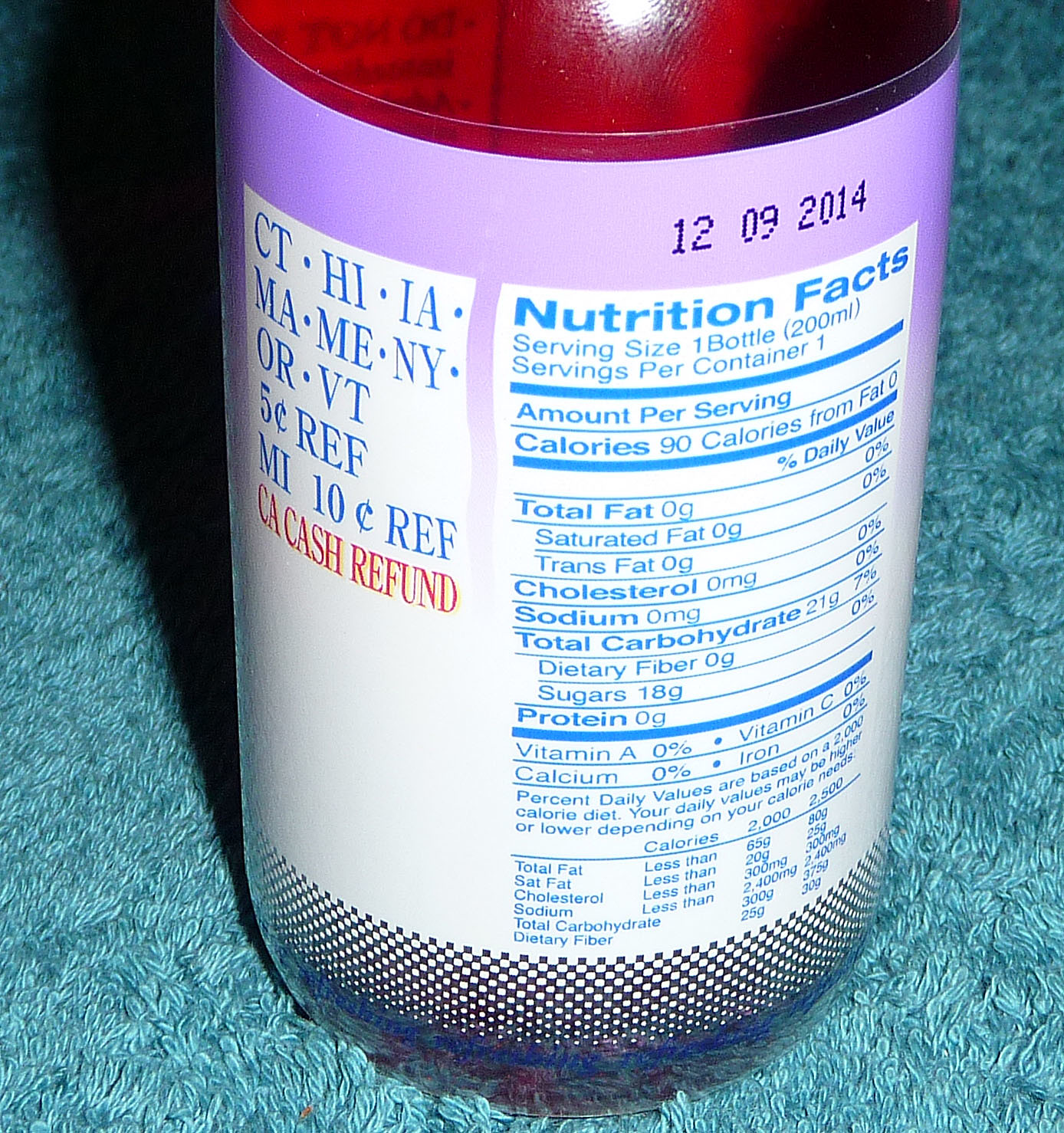This is a close-up photograph of a jar or bottle of a consumable liquid, prominently displaying its back label. The label itself blends shades of pink, lavender, and white, fading to white at the bottom. Positioned on a fuzzy, teal blue rug, the jar reveals its red contents through the semi-transparent material. The label details include nutrition facts such as 90 calories per bottle and 18 grams of sugar. It also lists various U.S. states with bottle recycling refund values: Connecticut, Hawaii, Iowa, Maine, Massachusetts, New York, Oregon, and Vermont offer a 5-cent refund, Michigan offers 10 cents, and California has a distinct cash refund. The expiration date clearly reads 12-09-2014.